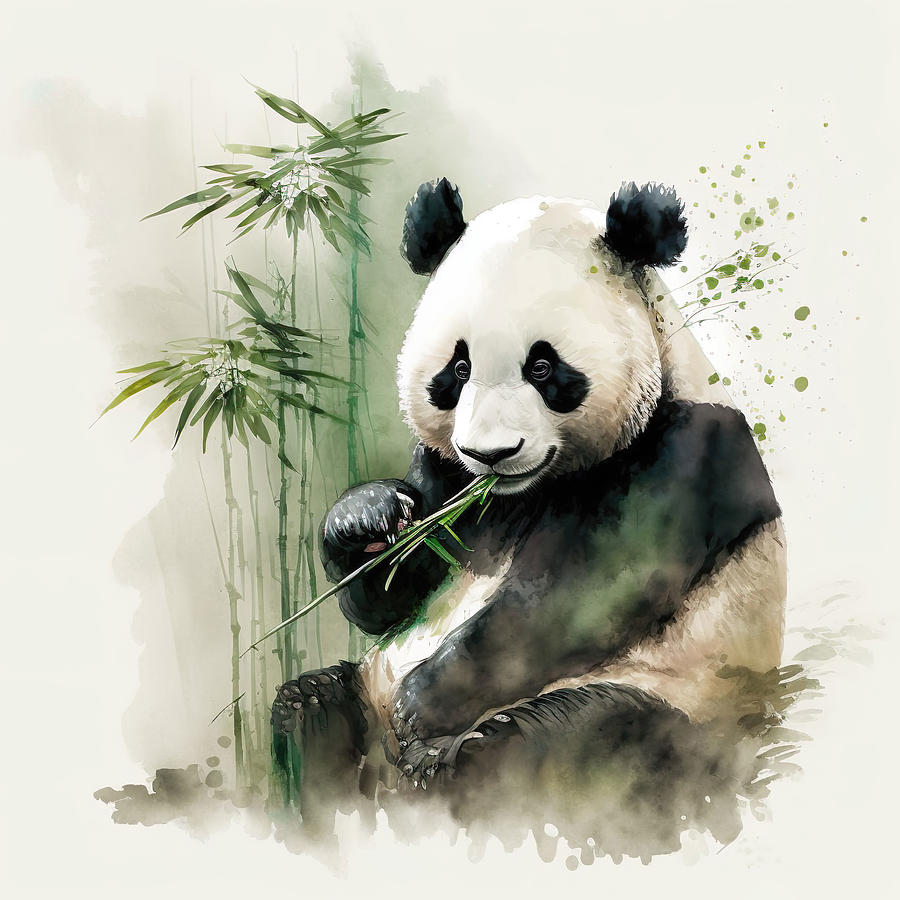This painting, combining elements of realism and watercolor, portrays a giant panda seated against a white background with subtle gray and green shading. The panda, characterized by its distinctive black ears, eye patches, limbs, and its white face, muzzle, and body, is vividly detailed with a bamboo stalk in its mouth. The watercolor technique gives its body a hazy, almost melty appearance, blending black, gray, and green tones. The panda is depicted sitting down, holding the bamboo with its feet up, and gazing toward the viewer. To the left, there are several bamboo stalks with leafy tops, adding a rich green contrast. Green splatters, possibly evoking movement or windblown foliage, decorate the top right corner, enhancing the dynamic and stylized feel of the piece.